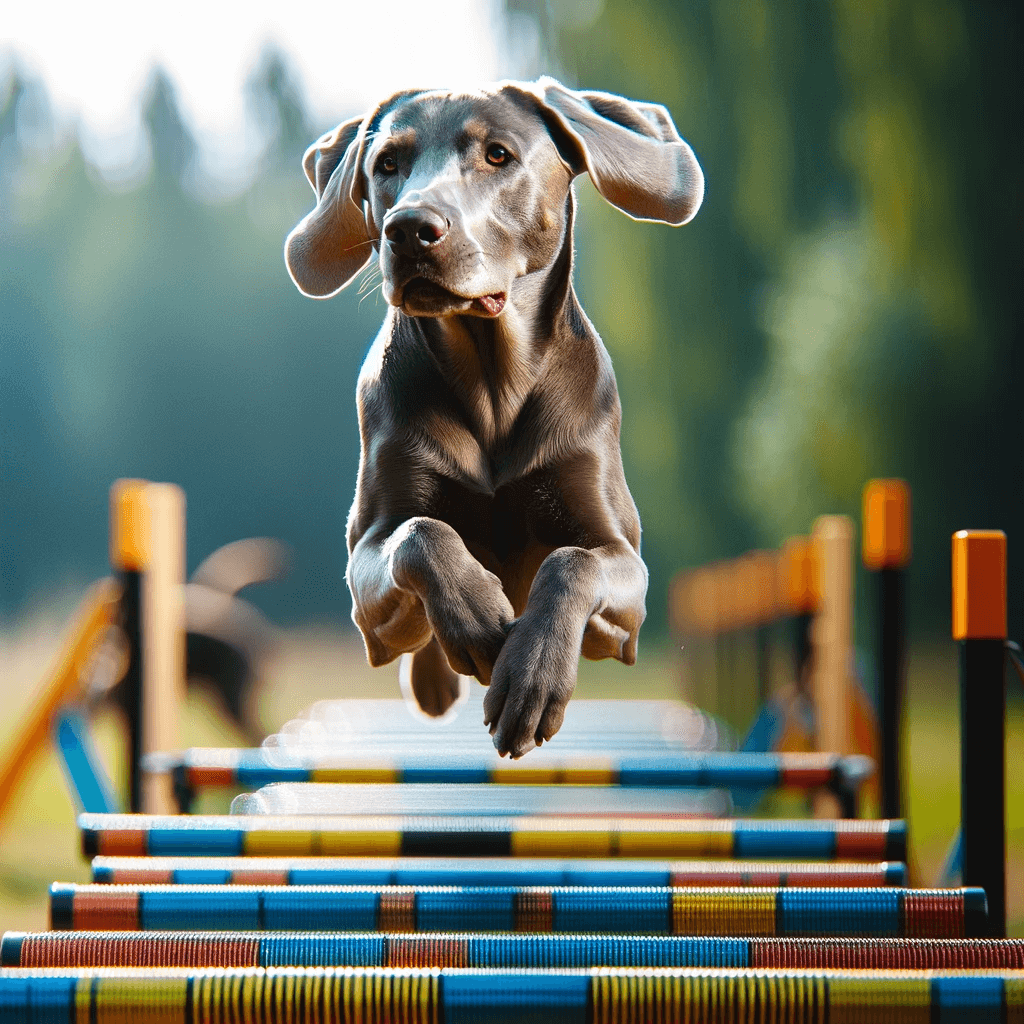In this square-shaped digital render, a medium to large brown dog is captured mid-leap as it navigates an obstacle course. The dog’s paws are positioned downwards as it soars through the air, giving a dynamic sense of motion. The fur of the dog gleams with an almost unrealistic shimmer, suggesting the use of AI-enhanced or computer-generated imagery. The dog is jumping over colorful striped poles in blue, yellow, and red, which are lined up below it. There are also black posts with orange sections along the sides, contributing to the orderly structure of the obstacle course. The background, a blur of green and blue hues along with indistinct trees, enhances the focus on the dog while suggesting an outdoor environment.